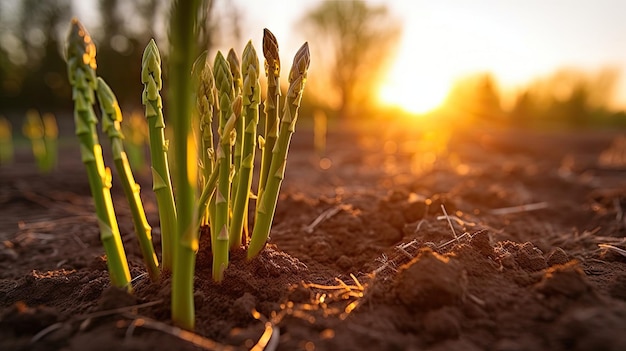This detailed photograph, taken from a low angle near the ground, captures a garden plot with freshly tilled brown soil. Emerging from the soil are vibrant light green asparagus sprouts, just beginning to bud and stand upright. The delicate shoots lack leaves and share the ground with a scattering of dry stems and debris. In the foreground, approximately ten asparagus spears are clearly visible, with additional sprouts fading into a blurry, out-of-focus background.

The setting sun near the horizon casts a radiant white and orange glow across the sky, contributing to the blurred, almost ethereal atmosphere. The background reveals a line of cypress trees and a wooden slatted fence, possibly intended to keep out animals. Despite its barrier, the fence seems porous enough for small creatures to navigate. This shallow depth of field emphasizes the sprouting asparagus while blending the distant elements into a diffuse backdrop, capturing the serene essence of this burgeoning garden environment.